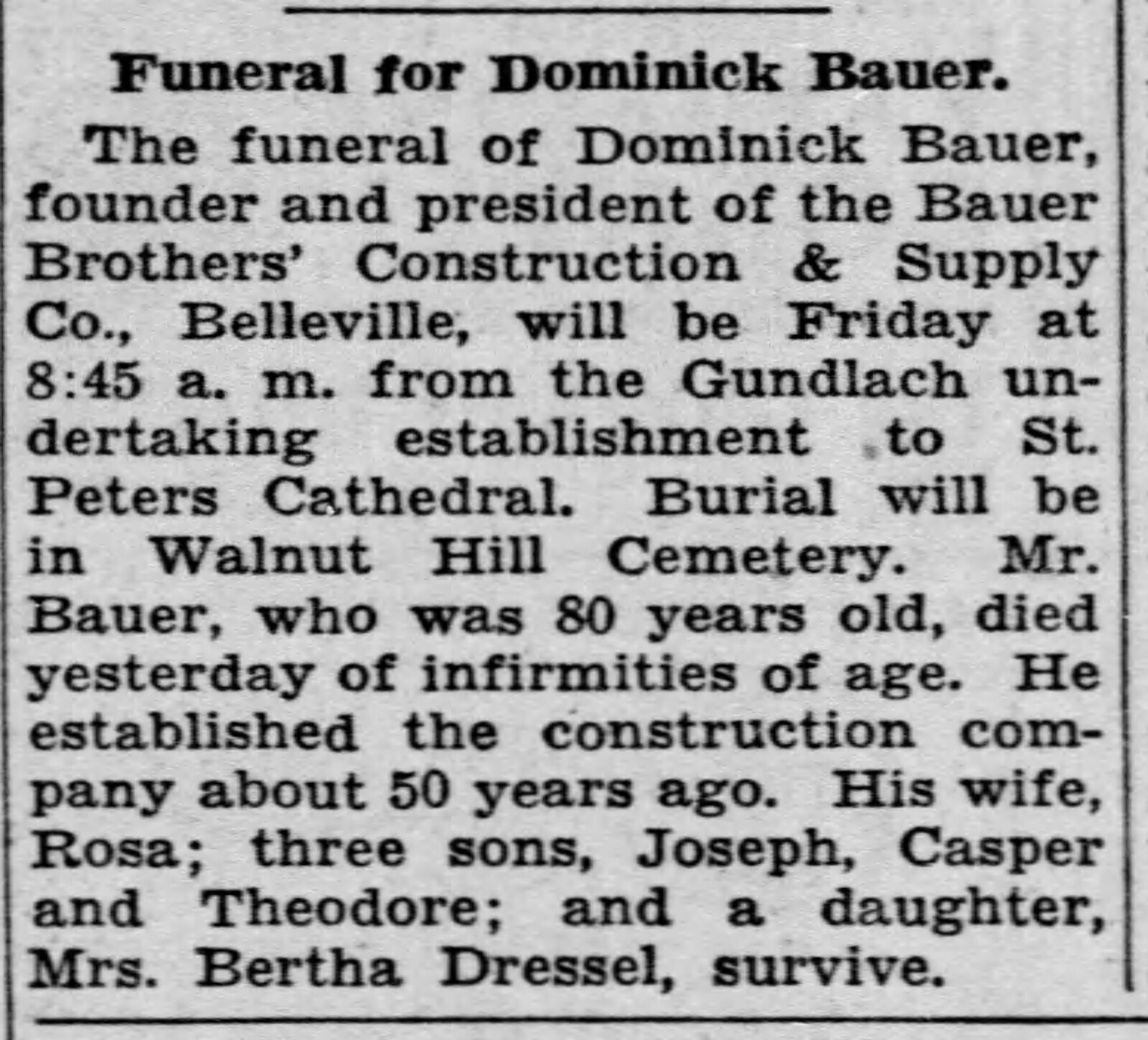The image is an excerpt from a newspaper featuring an obituary framed by a thin black border forming a square around the text. The background is light gray and the text is printed in black. The headline reads, "Funeral for Dominic Bauer." The article details that Dominic Bauer, founder and president of the Bauer Brothers Construction and Supply Company in Belleville, passed away at the age of 80 due to infirmities of age. His funeral will be held on Friday at 8:45 a.m. from the Gundlach Undertaking Establishment to St. Peter's Cathedral, with burial at Walnut Hill Cemetery. Bauer established his construction company approximately 50 years ago. He is survived by his wife, Rosa; three sons, Joseph, Casper, and Theodore; and a daughter, Mrs. Bertha Dressel.